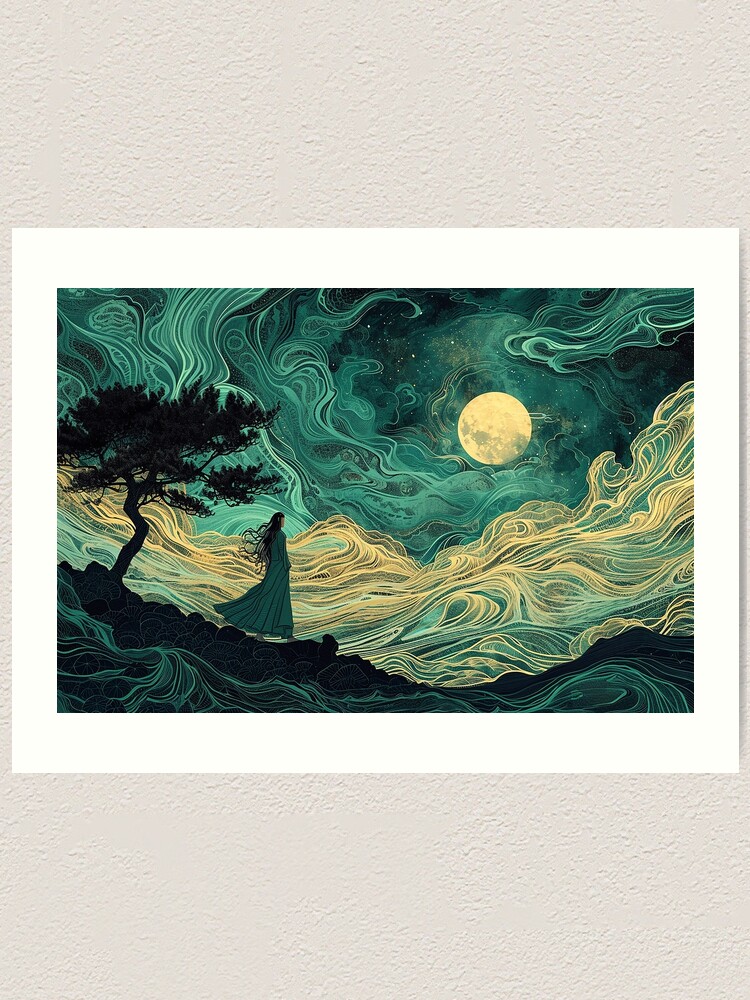This image depicts a moody, atmospheric painting framed in white and set against a light gray or cream-colored wall. The nighttime scene features a woman with long, flowing dark hair, dressed in a dark teal, turquoise, or white gown that reaches her knees, creating a striking contrast with the rocky ground beneath her. She is walking downhill to her left, near a small yet prominent black silhouette of a pine tree, which twists upward with intricate branches. The sky overhead is a swirl of green, yellow, and turquoise, with smoky cloud representations and possibly stars. Dominating the center right of the painting is a yellow moon, detailed with darker areas suggesting lunar seas. The background is filled with spiraling, dreamlike designs that blend into this surreal, almost artistic portrayal of a nighttime landscape. The entire scene is encased within a rectangular frame that enhances the fantastical and atmospheric qualities of this detailed and evocative artwork.